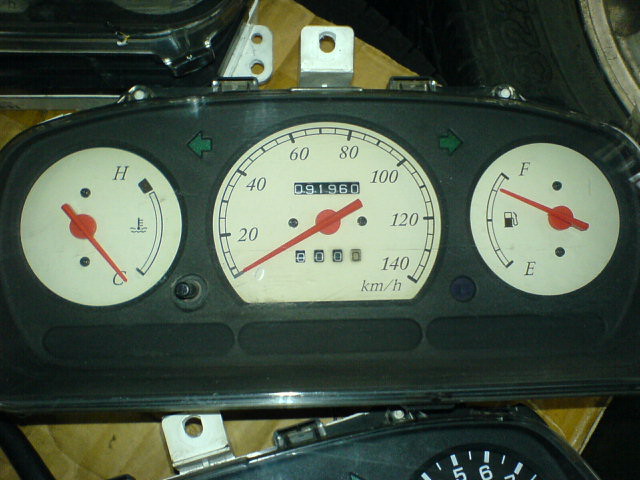A removed car dashboard, crafted from dark gray to nearly black plastic, is the focal point of this image. The dashboard, detached from its vehicle, is displayed atop a brown cardboard box. To the top of the dashboard are two green arrows, one pointing left and the other right. Centrally located are three white-faced gauges. 

On the left, the temperature gauge features a 'C' (cold) at the bottom and an 'H' (hot) at the top, with a red needle pointing towards the 'C'. The middle gauge is a speedometer marked in kilometers per hour, starting at 0 and increasing in increments of 20 up to 140. Both the trip meter and odometer read 0, with the latter showing a mileage of 091960. The red needle of the speedometer rests at the zero mark. To the right, the fuel gauge is segmented from 'E' (empty) to 'F' (full) in quarter increments, with a red needle indicating three-quarters full.

A silver metal bracket is affixed to the top of the dashboard, providing a point for mounting. Additionally, at the top and the bottom edges of the image, parts of other, similarly removed dashboards are visible though partially cut off from the frame, hinting at more instruments awaiting assembly or repair.